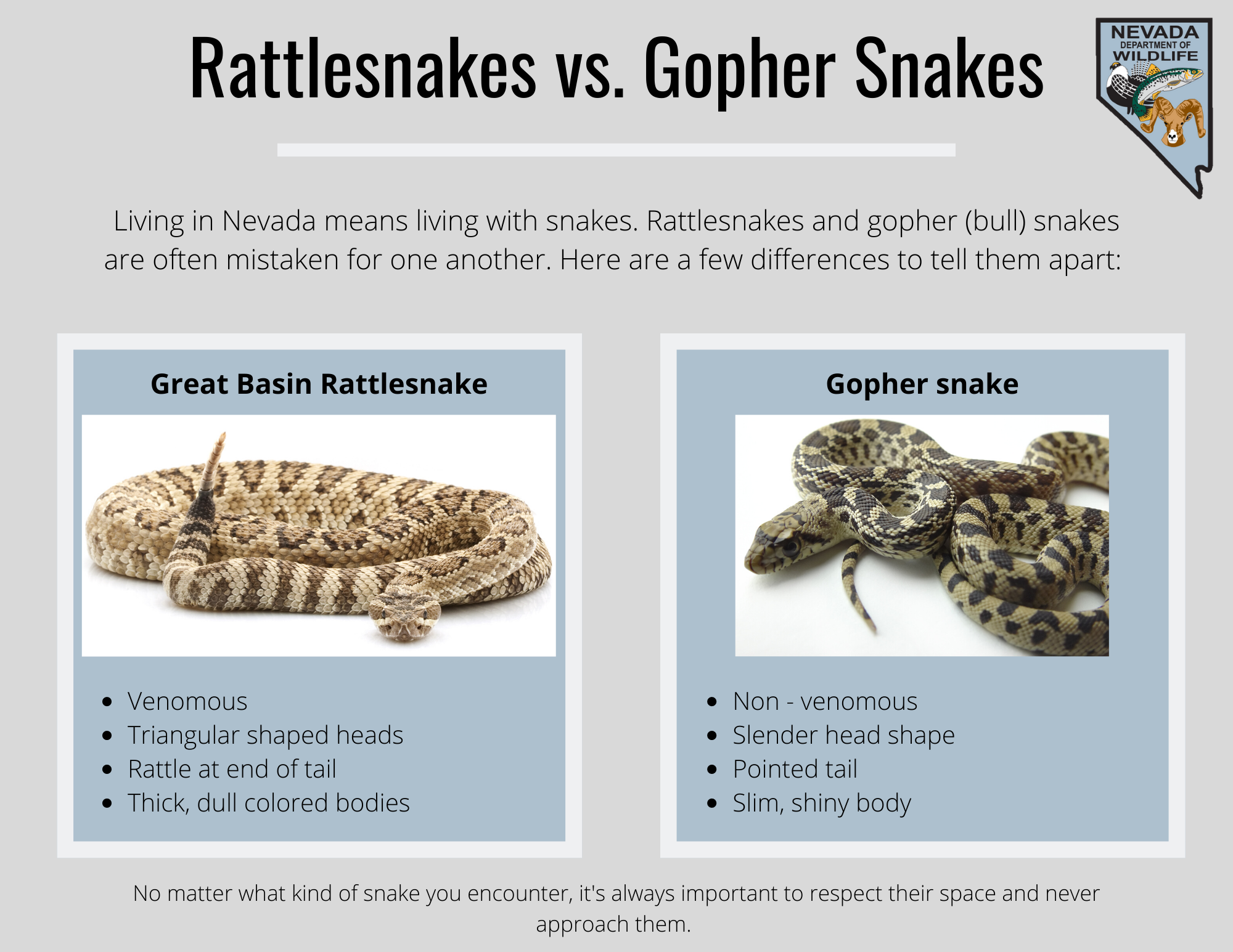The infographic illustrates the differences between rattlesnakes and gopher snakes, emphasizing that living in Nevada means living with snakes. The top header in bold black text reads "Rattlesnakes versus Gopher Snakes," followed by the statement, "Living in Nevada means living with snakes." Both species are often mistaken for one another, and the infographic provides key differences to help distinguish them. On the left, the Great Basin rattlesnake is featured within a blue-gray box; the snake has a light tan body with darker brown markings, a diamond-like pattern along its back, and dark brown stripes leading to its rattle. Captions describe it as venomous, with a triangular-shaped head, a rattle at the end of its tail, and a thick, dull-colored body. On the right, the gopher snake is also set within a blue-gray box, showing a greenish-gray body with dark blotches. It has a slender head shape, a pointed tail, and a slim, shiny body, and is identified as non-venomous. Each box includes the descriptive titles "Great Basin Rattlesnake" and "Gopher Snake" respectively. The top right corner displays the Nevada Department of Wildlife emblem, which includes images of a fish, a bird, and a bighorn sheep. The overall background of the infographic is gray. Beneath both snake images, a reminder advises, "No matter what kind of snake you encounter, it is always important to respect their space and never approach them."